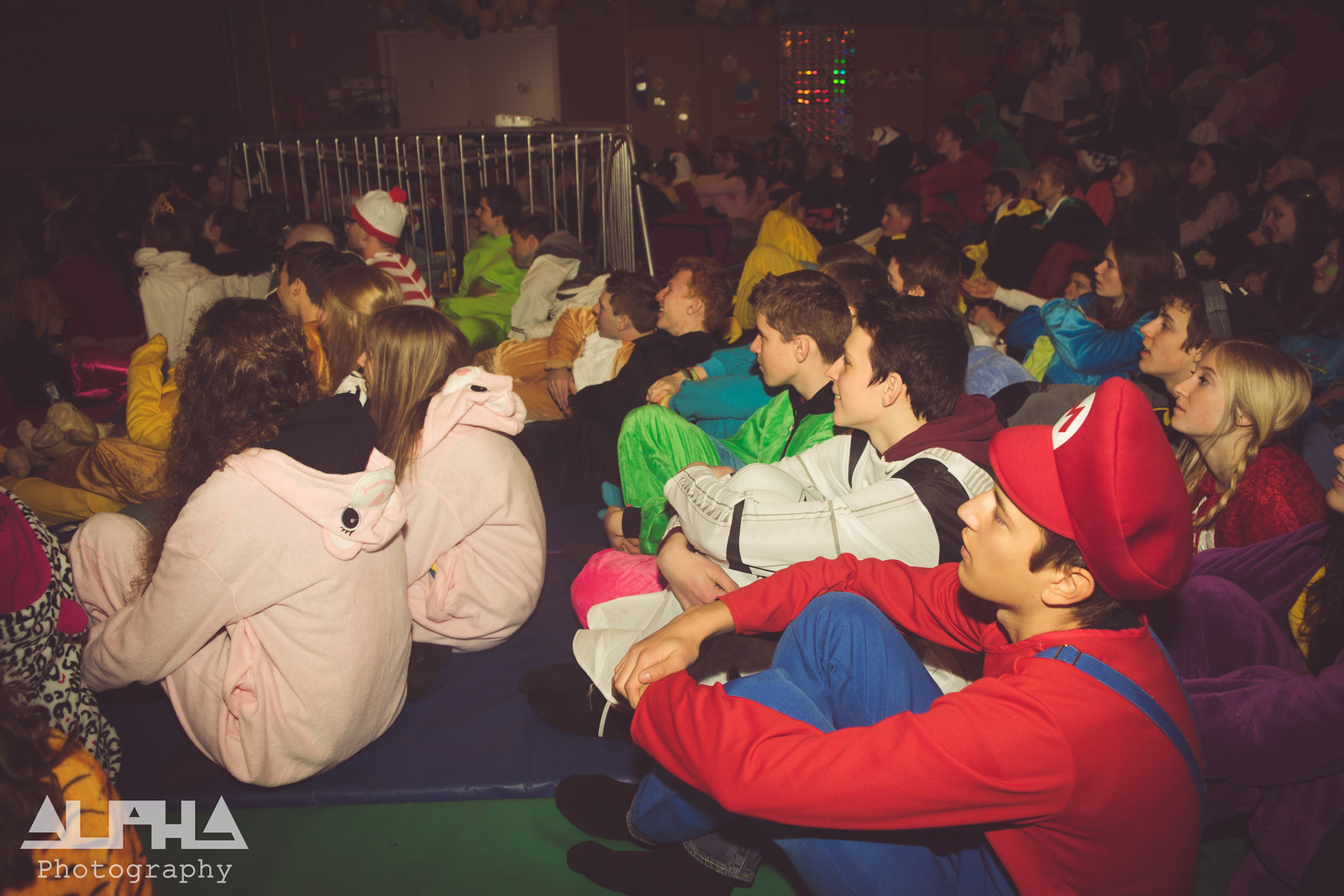The image depicts a large group of over 50 high school-aged students sitting cross-legged on a green floor with a blue mat in sections, likely participating in a Halloween-themed costume party or outdoor movie night. The scene is dimly lit, adding to the dark ambiance. All the individuals appear to be facing towards the left side of the image, engrossed in their activity. Costumes are a highlight, with visible characters including Mario in a red conductor hat and Where's Waldo in a red and white striped shirt. In the bottom left corner, two girls, around 15 years old, are wearing pink dog pajamas. The middle section of the image shows metal bars that resemble a gate or barrier, adding an element of intrigue. The photograph, attributed to "alpha photography" in white text at the bottom left, captures not just the costumes but also the layered seating arrangement, suggesting a slight incline towards the back right of the image.